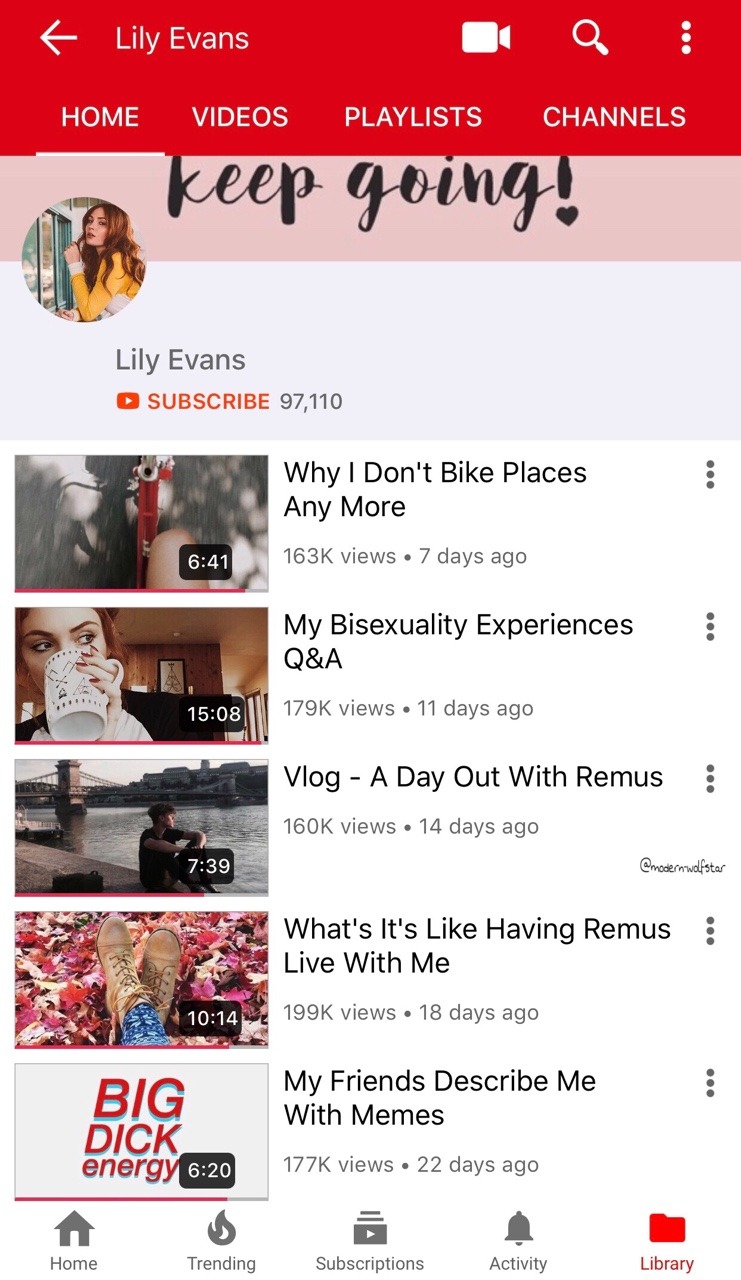The image displays the YouTube channel page of Lily Evans. At the top of the page, you can see various tabs including "Home," "Videos," "Playlists," and "Channels," with the "Home" tab currently selected. Dominating the screen is a picture of Lily Evans, a white woman appearing deep in thought while outdoors. She is wearing a yellow top, and next to her image is partially visible text featuring an exclamation point, starting with the words "keep going."

Lily Evans has amassed approximately 97,000 subscribers, showcasing her significant online presence. The screen also features previews of her five most recent videos. The latest video, titled "Why I Don't Bike Places Anymore," was uploaded seven days ago. Other videos include "My Bisexuality Experiences Q&A," "Vlog: A Day Out with Remus," "What It's Like Having Remus Live with Me," and "My Friends Describe Me with Memes."

Each video is represented by a thumbnail image, with the last video displaying the phrase "big dick energy" and having a duration of six minutes and twenty seconds. The remaining videos have slightly longer run times, with "My Bisexuality Experiences Q&A" being approximately fifteen minutes long.